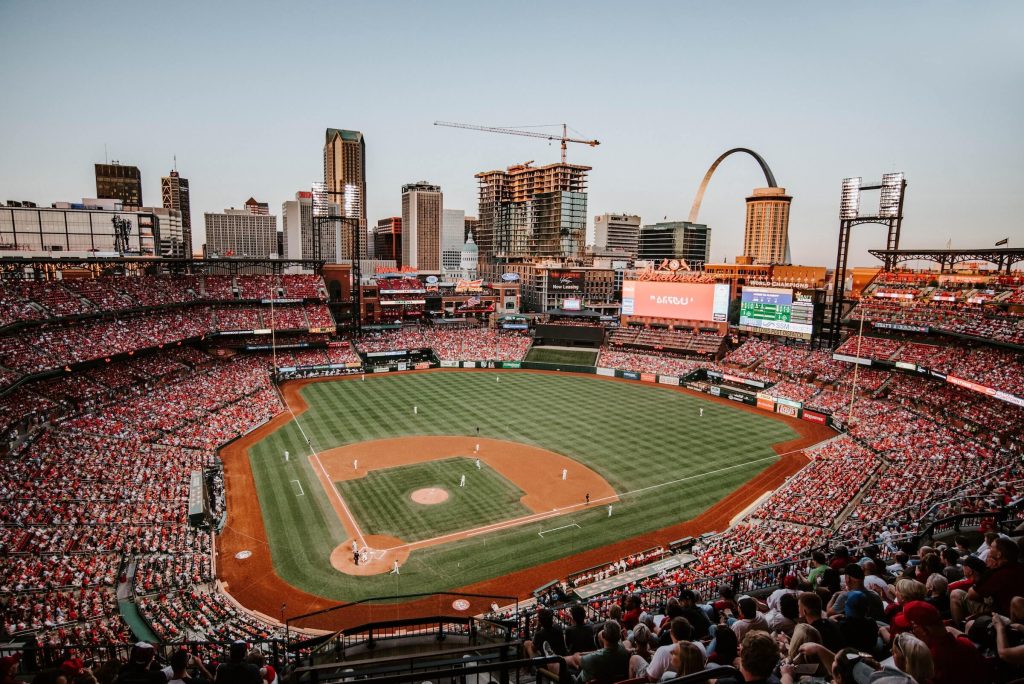The photograph captures a bustling baseball stadium, packed with spectators, many donned in red, creating a vibrant sea of color. The overall image is rectangular, with the longer sides at the top and bottom. At the center lies a meticulously maintained, triangular-shaped field with a striking green grass pattern, with the home plate positioned towards the bottom left. Encircling the grassy area is a border of dark brown dirt, followed by a low wall and tiered seating that ascends like steps, bringing higher seats further away from the field. The vantage point appears to be from within the stands, offering a closer view of the fans nearer the bottom of the image. Above the middle of the image rises a city skyline with numerous skyscrapers, some under construction, and on the right side, the iconic St. Louis Arch stands prominent against the light blue sky.